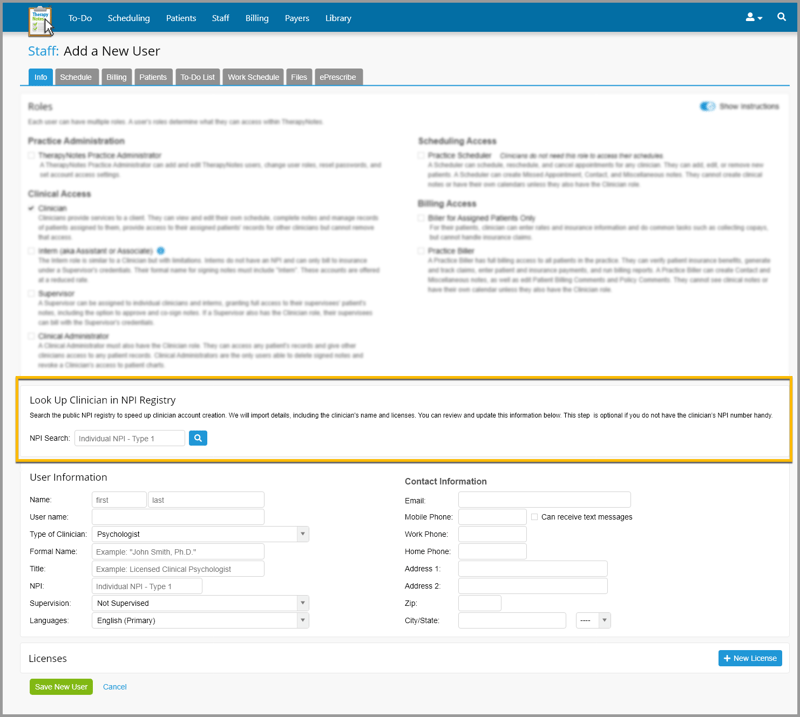In the image, we observe what appears to be a web interface displayed on a desktop screen. At the top right corner, there’s a white magnifying glass icon for search functionality, accompanied by a white, human-like figure emblem which likely represents a user profile. Adjacent to this user profile icon is a downward-pointing arrow, suggesting a dropdown menu.

On the top left corner, there's an image depicting a writing area, complete with a mouse cursor. Running horizontally across the top, we see a navigation menu with the following options: TO DO, SCHEDULING, PATIENTS, STAFF, BILLING, PAYERS, and LIBRARY.

Immediately below the picture, the words "STAFF" and "ADD A USER" are visible, hinting at user management functions. Further down, another horizontal menu offers additional sections: INFO, SCHEDULE, BILLING, PATIENTS, TO DO LIST, WORK SCHEDULE, FILES, and PRESCRIBE. Unfortunately, part of this area is obscured, rendering some text unreadable.

In the bottom half of the image, there is a prominent yellow rectangle stretching across the width of the image, containing the words "LOOK UP," "CLINICIAN," and "NPI REGISTRY." Below this, there’s a user information form where various user details such as name, username, and title can be entered.